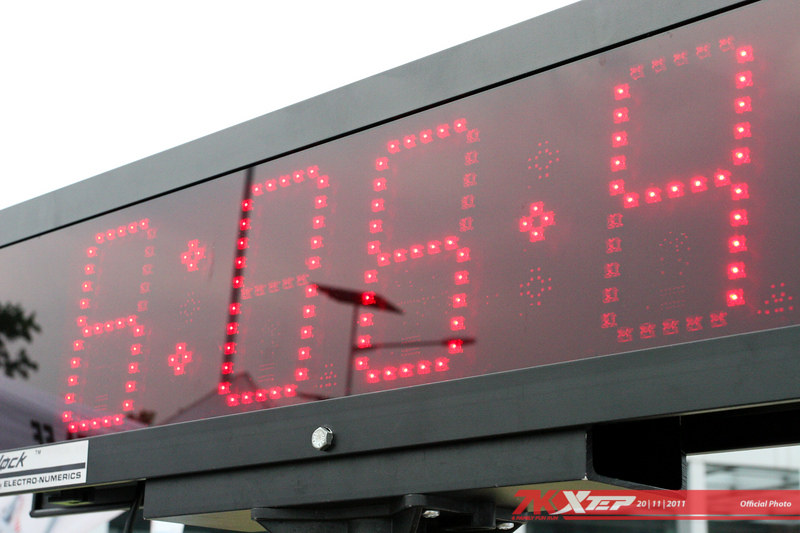This image shows a sleek, long rectangular digital clock. The clock features a minimalist design with a black frame and vibrant red LED lights forming the numerical display. The current time shown is "6:06" with an additional "+9" seconds indicator, distinguished by individually lit red dots for precision. In the bottom left corner of the clock's frame, there is a contrasting white rectangle with black text that reads "electric numbers". Towards the bottom right of the frame, a long red rectangle can be found, containing the text "7k" beside it, and overlayed on the rectangle in white text is the notation "XEP 20/11/2011 official photo". This detailed composition underscores the clock's modern digital aesthetic and functional clarity.